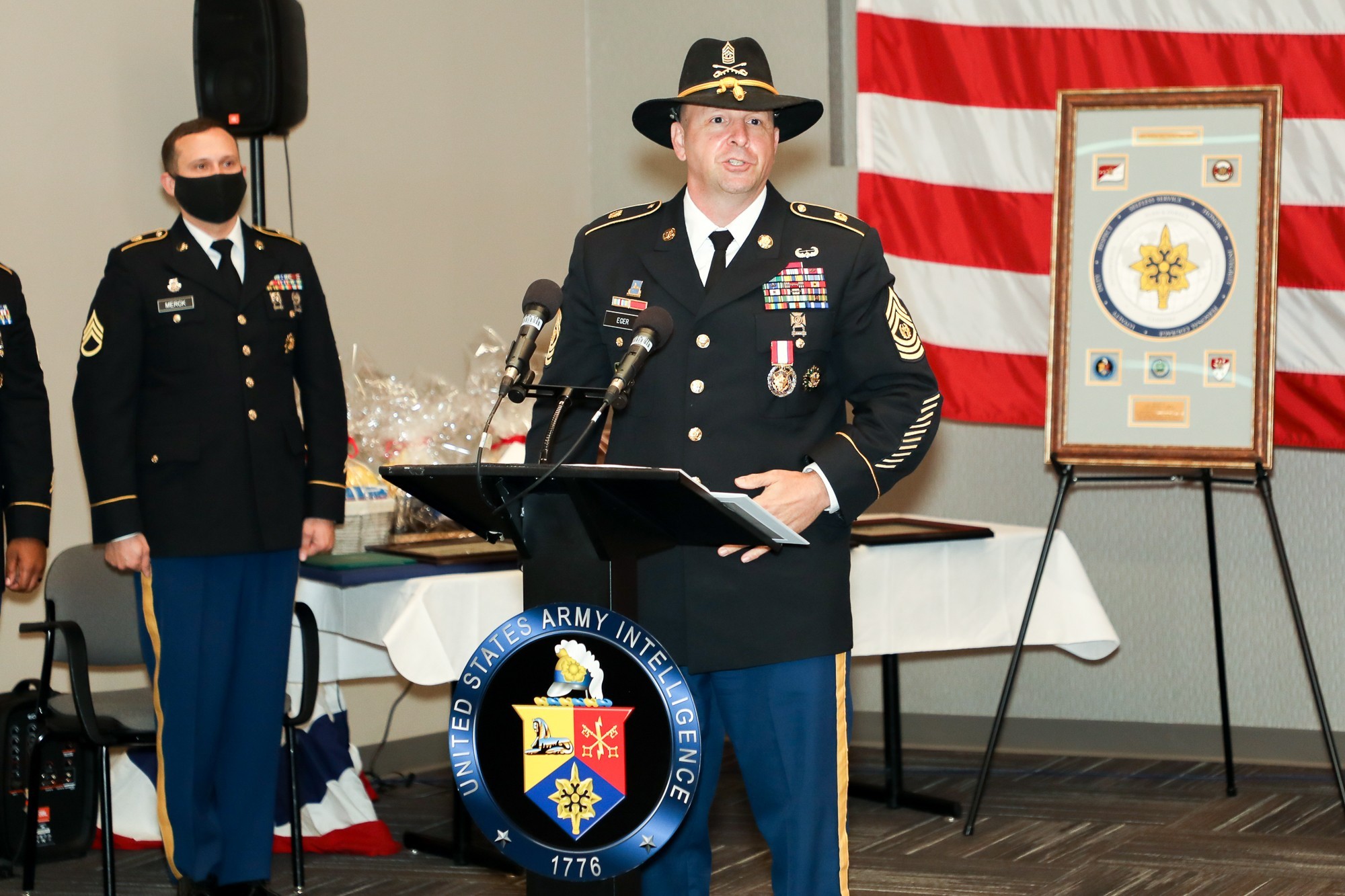The image captures a formal military event, possibly a speech or intelligence briefing. At the center is a U.S. Army sergeant standing behind a small podium with three microphones. The podium features a circular emblem with the text "United States Army Intelligence, 1776" and a coat of arms in the middle, divided into yellow, red, and blue sections resembling an upside-down arrow with an object on top. The sergeant is in full dress uniform, including a dark blue jacket adorned with medals, a white shirt, a black tie, blue pants with a yellow stripe, and a cavalry-style hat. To the left of the podium stands another soldier in a similar military outfit, wearing a black mask. Behind them, part of an American flag is visible, along with a three-legged support for a large picture that has a diamond and some other indistinct details. The floor is made of wooden tiles, contributing to the formal atmosphere of the scene.